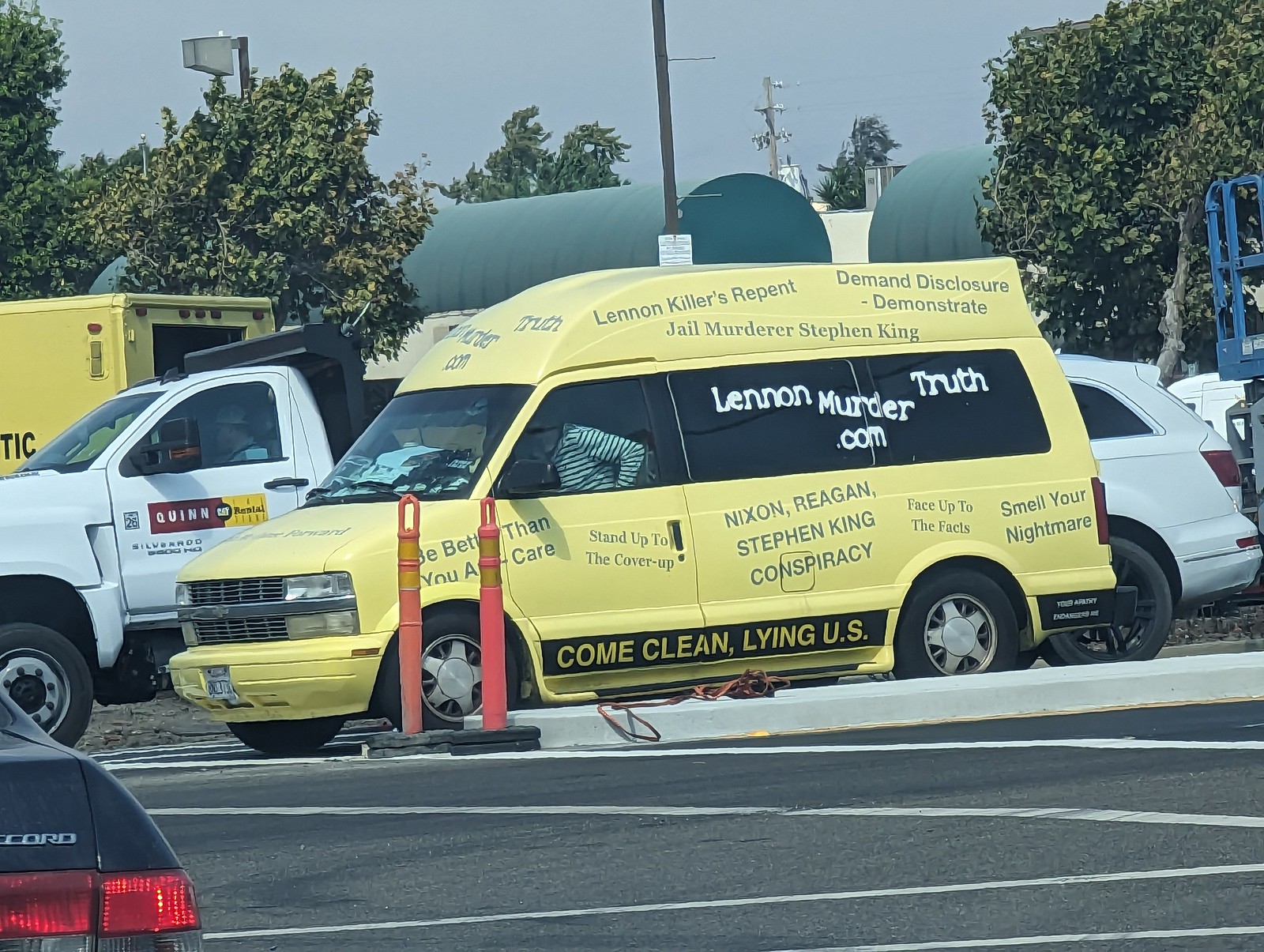This color photograph captures a busy parking lot scene centered around a conspicuous yellow van adorned with a series of provocative statements. The van, which features phrases like "Lennon killers repent," "Jail murderer Stephen King," "Nixon Reagan Stephen King conspiracy," "Smell your nightmare," and "Face up to the facts," also includes the website "LennonMurderTruth.com" and the plea "Come clean lying U.S." In the foreground, the corner of a black Honda Accord's trunk is visible. A woman, clad in a white and black striped long-sleeved shirt, sits in the driver's seat of the yellow van. Nearby, two orange traffic cones frame the controversial vehicle. Surrounding the van, several other cars are parked, including a white car, a white truck, and a yellow truck. Beyond the parking lot, trees punctuate the landscape, with an industrial area featuring large tanks, an electric lift, light poles, and various infrastructural elements adding depth to the background.